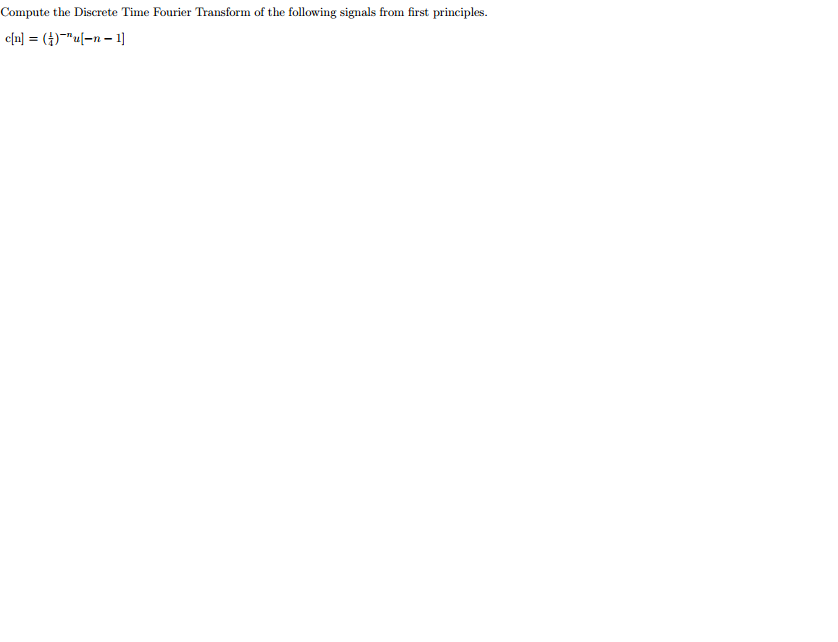A problem statement is displayed asking to "Compute the Discrete Time Fourier Transform of the Following Signals from First Principles." The text is capitalized with the initial letter of each word starting with a capital. Below this instruction, the given signal is presented as:

c[n] = (1/4)^-n * u[-n - 1]

Here, "c[n]" is enclosed in square brackets and followed by an equal sign. Within the expression, there is a fraction "(1/4)" raised to the power of "-n," followed by "u," which is accompanied by "[-n - 1]" in square brackets. The notation for "-n" and "u" appears in a smaller, italicized font. The rest of the image is filled with white space.